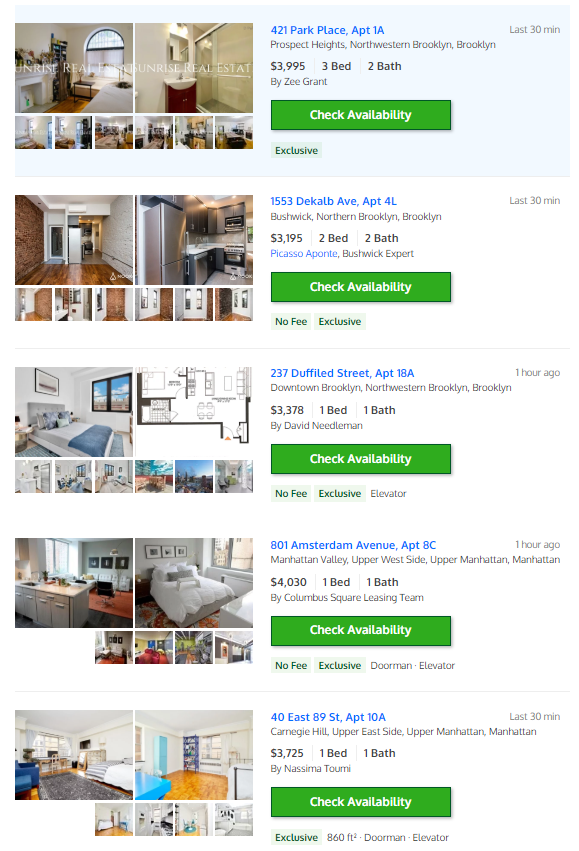Screenshot of a rental properties app showcasing five available options in New York City. The interface prominently features two main property photographs with six additional thumbnails beneath each, except for the bottom two listings which have four thumbnails justified to the right. 

Each property listing includes a bright green "Check Availability" button, detailed information such as addresses, contact details, prices, and apartment specifications. 

- **Listing 1:** 
  - **Address:** 421 Park Place, Apartment 1A, Prospect Heights, Northwestern Brooklyn, Brooklyn.
  - **Price:** $3,995 per month
  - **Specifications:** 3 bedrooms, 2 bathrooms
  - **Posted by:** Z Grant

- **Listing 2:**
  - **Location:** Brooklyn
  - **Price:** $3,195 per month
  - **Specifications:** 2 bedrooms, 2 bathrooms

- **Listing 3:**
  - **Location:** Brooklyn
  - **Price:** $3,378 per month
  - **Specifications:** 1 bedroom, 1 bathroom

- **Listing 4:** 
  - **Location:** Brooklyn
  - **Price:** $3,000 per month
  - **Specifications:** 1 bedroom, 1 bathroom

- **Listing 5:** 
  - **Address:** 801 Amsterdam Avenue, Apartment 8C, Manhattan
  - **Price:** $4,030 per month
  - **Specifications:** 1 bedroom, 1 bathroom

- **Listing 6:** 
  - **Address:** 40 East 89th Street, Apartment 10A, Manhattan
  - **Price:** $3,725 per month
  - **Specifications:** 1 bedroom, 1 bathroom

Highlighted is the premium cost of living in New York City, with detailed insights into each rental option.